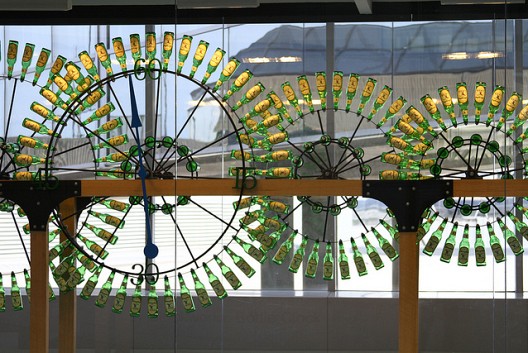The photograph, taken in landscape orientation, features a meticulously crafted wooden and black metal structure situated in an indoor setting. Prominently, the structure consists of wooden planks running horizontally, fastened together with black metal joints. Vertical wooden beams extend from these joints towards the floor. Attached to this wooden framework are four large, black wrought iron circles resembling the spokes of giant wheels or bicycle wheels. Each circle is adorned with empty green bottles, likely beer bottles with yellow labels, arranged in a continuous pattern around their perimeters. 

The largest circle, positioned to the left, doubles as a timepiece, featuring black numbers: 60 at the top, 30 at the bottom, 15 on the right, 45 on the left, with blue clock hands pointing to these markers. The other three circles, progressively smaller and to the right, lack any numerical markings or clock hands.

This entire assemblage is foregrounded by a yellow and black safety rail, adding a layer of industrial contrast. Beyond this intricate display, a large picture window reveals an outdoor scene with sunlight filtering through, highlighting the glass bottles. The reflection of a nearby building, characterized by a tan facade and a blackish roof with visible beams forming an A-frame, can also be discerned through the glass, adding to the depth and realism of the composition. The overall style of the image is a striking example of photographic representationalism realism.